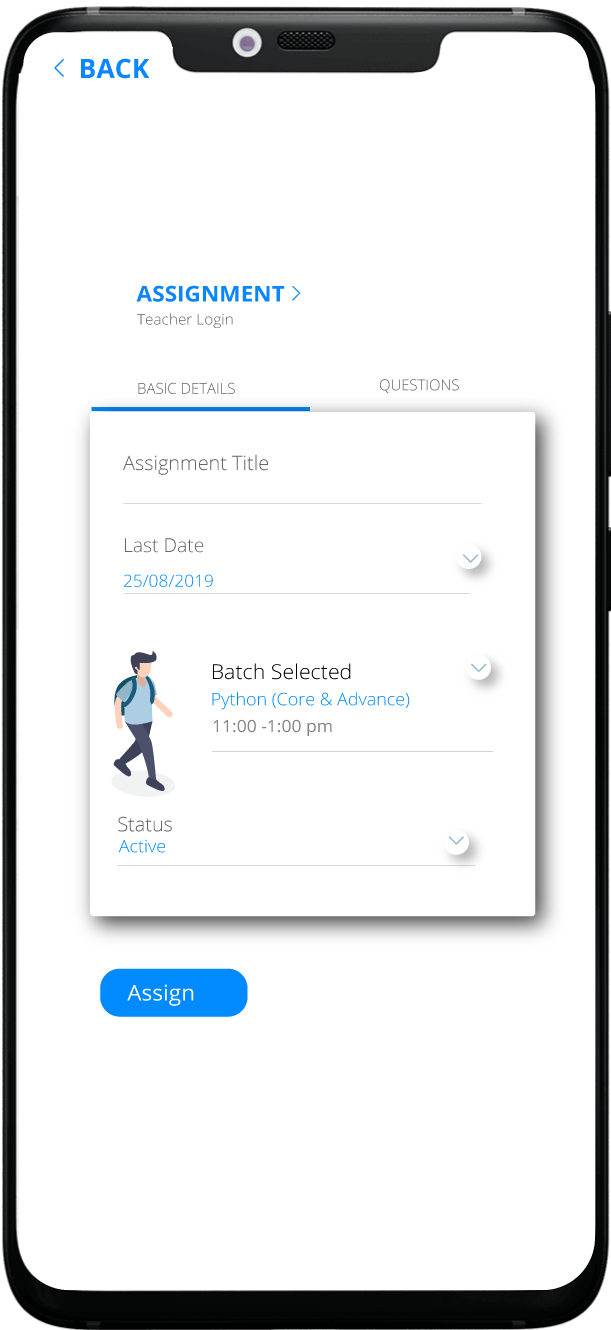The cell phone screen displays an interface for a teacher's login to an assignment management platform. At the top left, a small blue arrow points left next to the word "BACK" in uppercase letters. Just below, in bold blue text, is the title "ASSIGNMENT." Further down, in light gray, is the "TEACHER LOGIN" section.

On the left side of the screen, underlined in blue, is the label "BASIC DETAILS." Adjacent to it on the right is the word "QUESTIONS," followed by a square labeled "ASSIGNMENT TYPE." Below this header is "LAST DATE," showing "25-08-2019."

There is an animated image of a student wearing a blue shirt and a hat, carrying a book bag, walking. Beside this image, the text "BATCH SELECTED" appears in blue, detailing "PYTHON, CORE, AND ADVANCED, 11-1 PM." 

Further below, the status is indicated as "ACTIVE" in blue. The caption concludes with a horizontal blue oval button at the bottom, displaying the word "ASSIGN" in white uppercase letters.